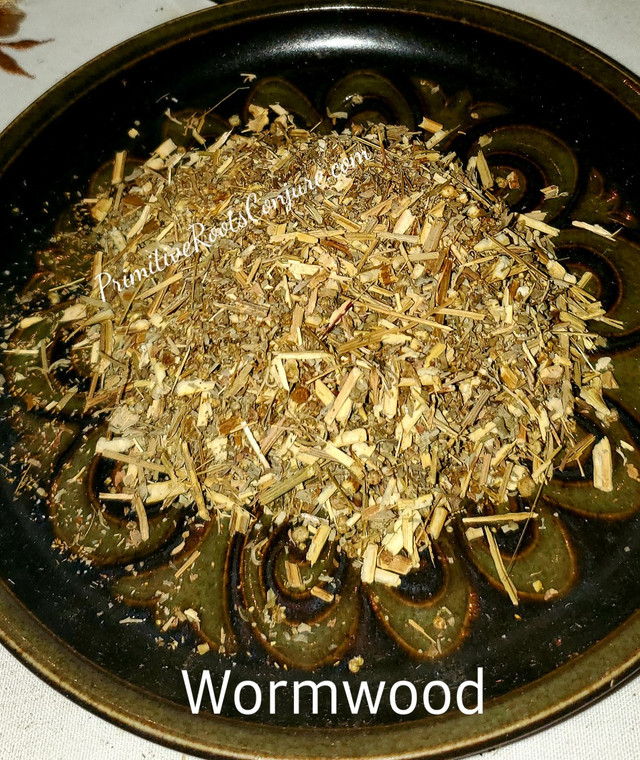The photograph features a black ceramic plate adorned with an olive green ring along its edge. The plate is topped with a scattered pile of wood chips in varied shades of tan, light brown, and yellowish-brown. Though partially obscured by the wood chips, the plate's center boasts a looping or circular design. The plate rests on a table draped with a tablecloth, possibly decorated with floral patterns. Curved cursive text across the wood chips reads "primitiverootsconjure.com," while bold white text at the bottom of the image states "WORMWOOD."